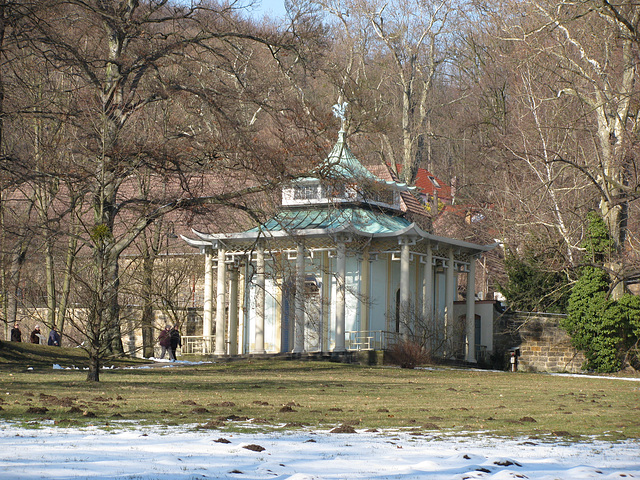The image focuses on an ornamental, oriental-inspired building positioned centrally in an outdoor setting during wintertime. The square building is characterized by significant architectural details, such as large circular pillars that wrap around its front and sides, and a triangular roof with eaves that curve upwards at each corner. A cupola with windows and a statue crowning the top add to its intricate design. Surrounding the building, the ground is lightly covered with snow, indicating the wintry season. To the right of the building, a brick wall is visible, while to the left, people are walking. The background is dominated by trees, and a grassy lawn area lies in front of the structure. The color palette includes shades of brown, green, white, light blue, and a touch of turquoise and red, with no text present in the image.